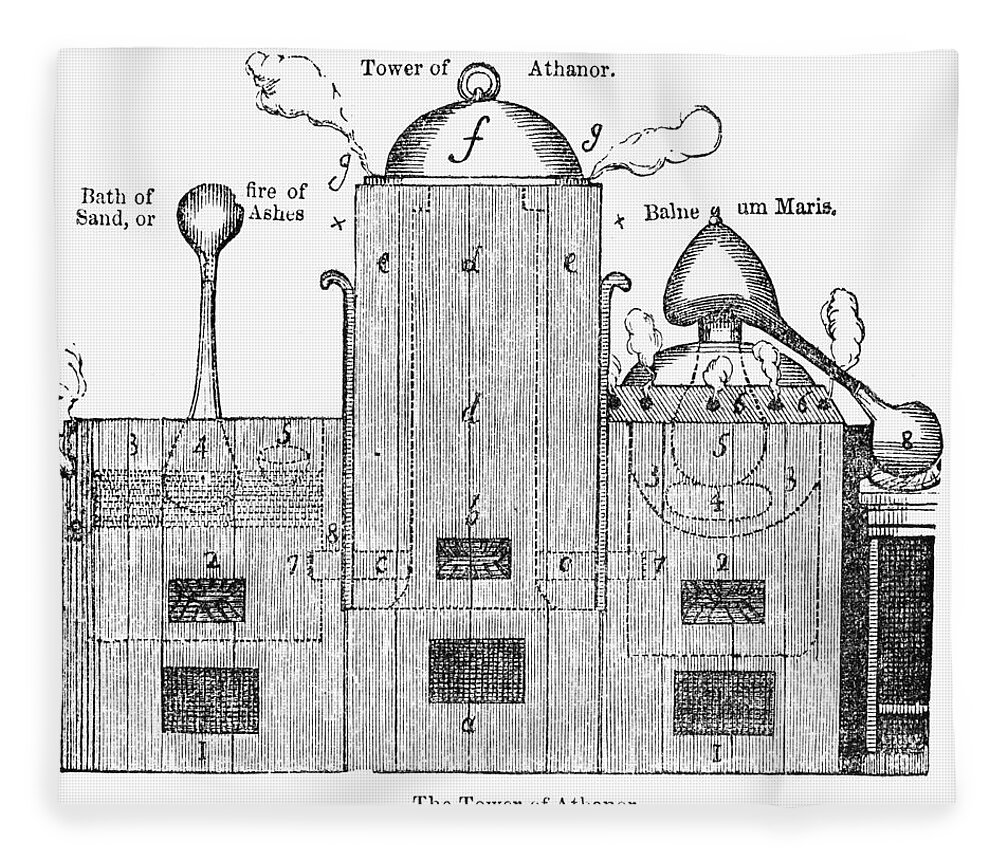The illustration is a black and white, old-fashioned diagram of a mysterious structure known as the Tower of Athanor, which appears to be a type of furnace or distillery. The drawing shows a side view of the tower, consisting of three main rectangular sections stacked vertically. The left rectangle has an elongated, pipette-like structure with a balloon-shaped top, and is labeled "Bath of Sand or Fire of Ashes." The central section of the tower features a prominently domed top with a ring at its tip and emits clouds of steam or smoke; it bears the name "Tower of Athanor." The right section is marked "Bonne Maris" and also has a dome with smoke emanating from small holes. The entire image is annotated with black font and various numerical labels designating different areas, contributing to its intricate, antiquated appearance.